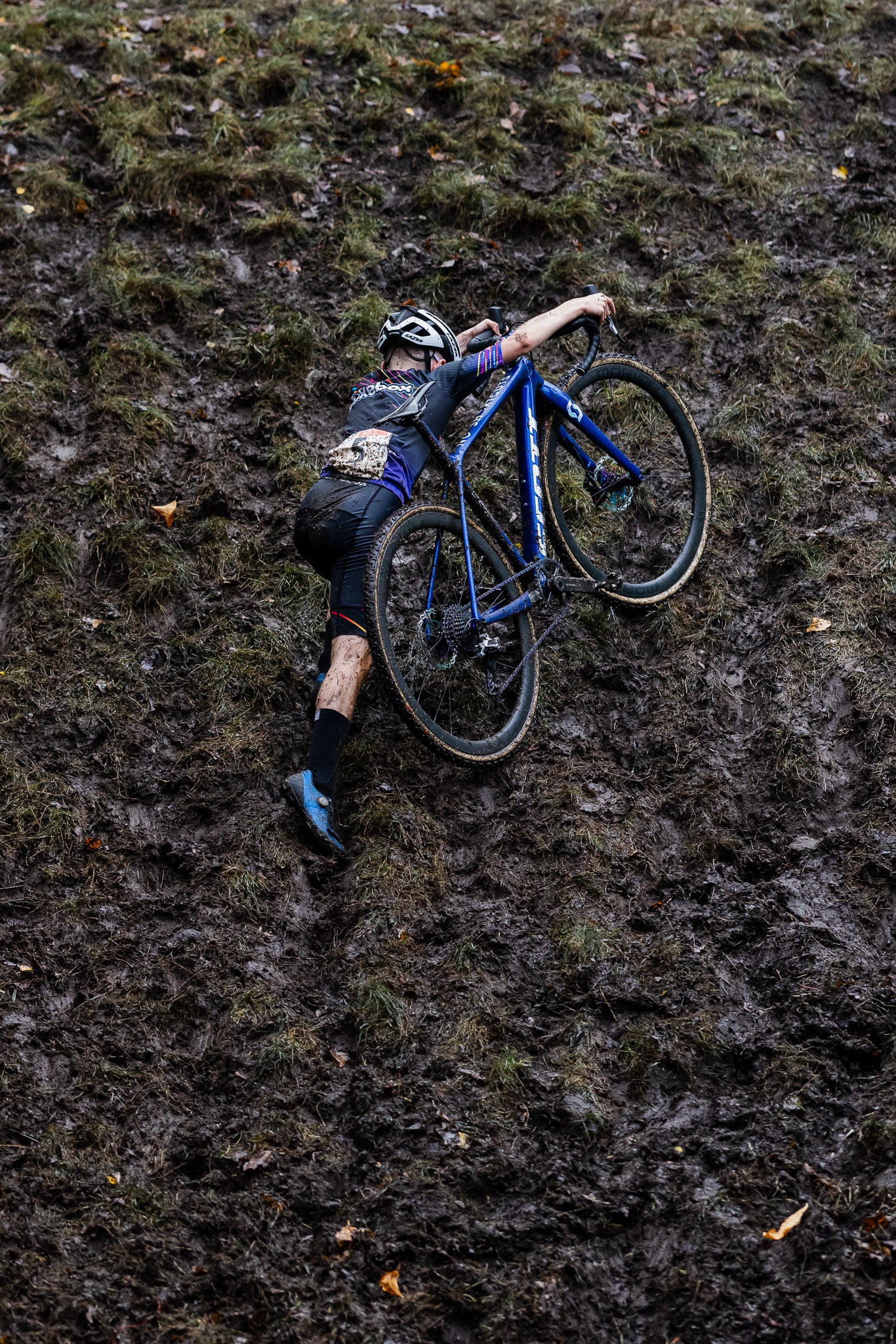In the image, a young mountain biker, likely an adolescent, is captured struggling up a steep, muddy hill. The backdrop is a mix of dirt and patches of green, indicating it could be spring or fall, possibly right after a rain shower. The scene is filled with ruts and wet, dark mud that splatters onto the biker’s exposed legs and dirties his uniform. The biker sports a predominantly dark outfit, featuring black shorts and a shirt that appears a mix of black, blue, and perhaps a hint of purple. He wears a black and white helmet, black socks, and blue and black shoes. His mountain bike, decorated in dark blue, bears a flat bar typical of professional mountain bikes. The young biker is positioned to the left of his bike, hands gripping the handlebars as he navigates the challenging terrain. A number "5" is visible on his back, suggesting he might be in a competitive event. The phone camera captures the muddy struggle in vivid detail, emphasizing the rider's effort and the tough trail conditions.